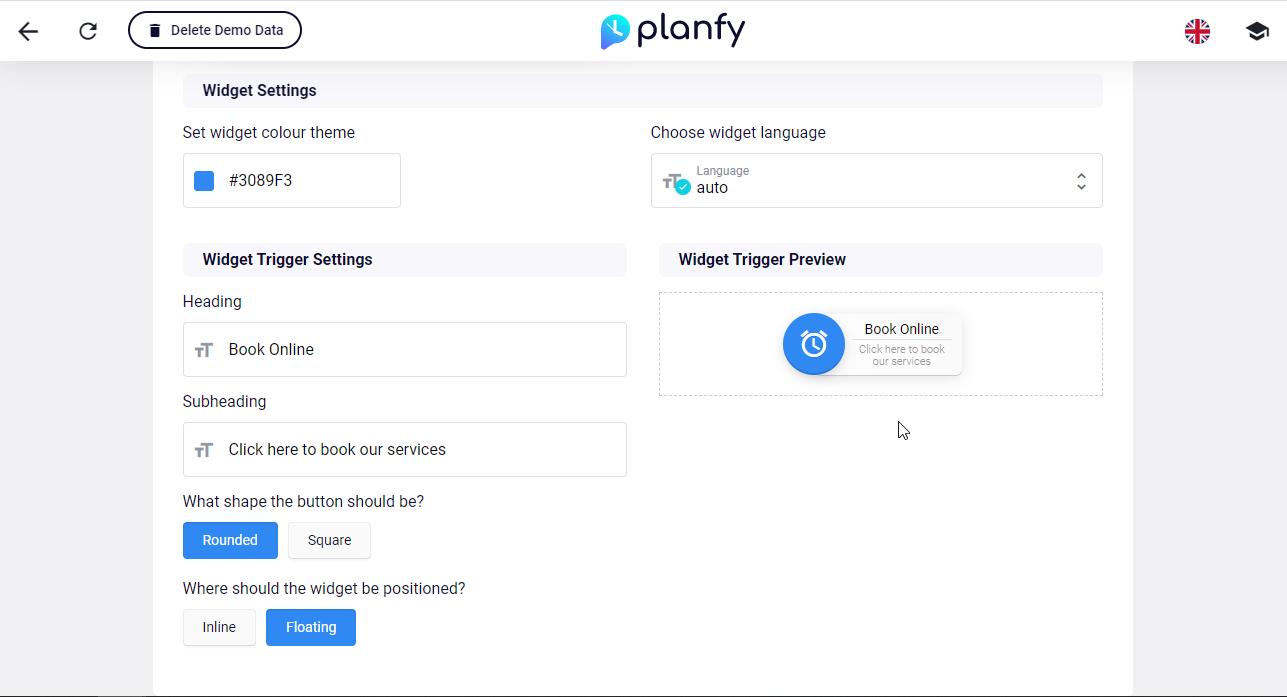This image is a detailed screenshot of a configuration interface within PLANFY, an online booking and scheduling platform. At the top of the interface, you can see the navigation controls featuring a left-pointing arrow, a refresh button, and an option to delete demo data. Centrally placed is the PLANFY logo, flanked on the right by a button that displays a British flag with a graduation cap icon.

Just below this navigation bar, the title "Widget Settings" is prominently displayed, alongside the subheading "Set Widget Colour Theme," which uses the British spelling of "colour." A medium royal blue shade, designated by the hexadecimal code #3089F3, is selected for the widget's color theme.

Following this, the interface provides an option titled "Choose Widget Language," which includes a drop-down menu where "auto" is the current selection.

On the left side of the screenshot, under "Widget Trigger Settings," several specific configurations can be seen:
1. The widget heading is set to "Book Online."
2. The subheading option reads "Click Here to Book Our Services."
3. The shape of the button is set to "Rounded," which is highlighted in blue.
4. The widget's position is configured as "Floating," also indicated in blue.

Towards the right-hand side, there is a section labeled "Widget Trigger Preview." This section displays a preview button with the title "Book Online" and the subheading "Click Here to Book Our Services."